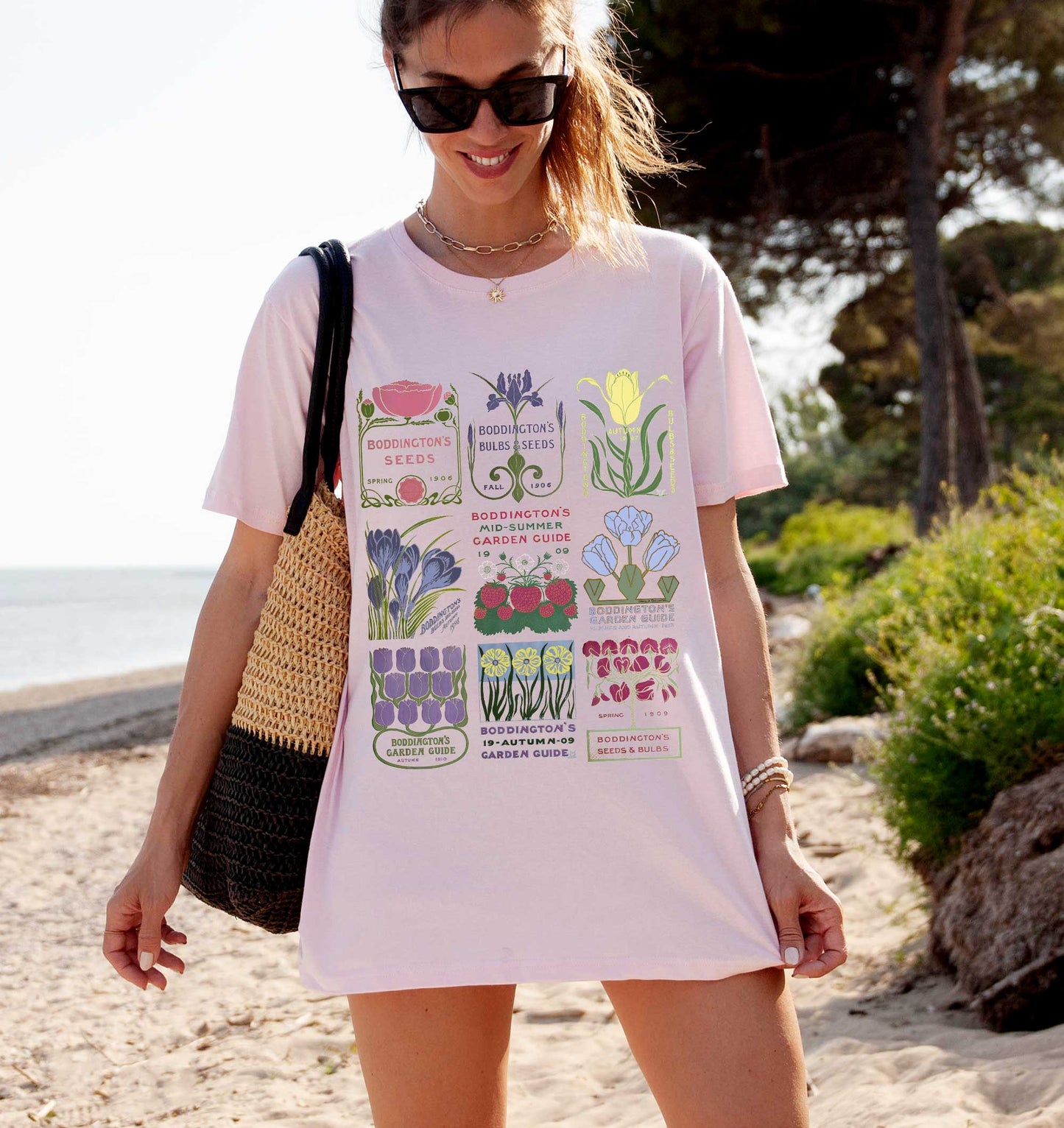The image features a smiling woman with blonde hair pulled back into a ponytail, wearing large black sunglasses. She dons a white, knee-length T-shirt adorned with pastel-colored flowers arranged in three distinct rows, each accompanied by small, unreadable text. Around her neck is a silver necklace, and she has bracelets on one wrist. Over her right shoulder, she carries a tan and black tote bag. The background reveals a sunny beach scene with light-colored sand or soil, accompanied by shrubs, tropical trees, and a glimpse of the blue ocean water on her left.